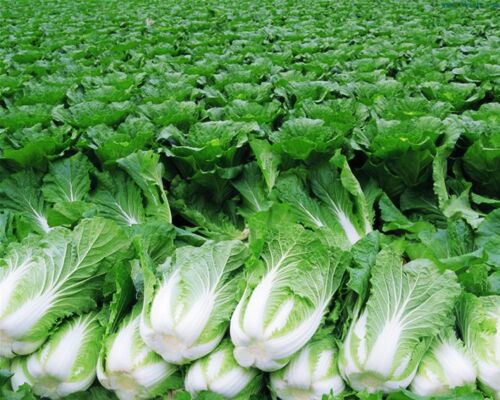The image depicts a vast, lush field of uniform, dark green cabbage plants, so dense that the ground is completely concealed beneath their thick leaves. In the foreground, some cabbages have been harvested, revealing their sturdy, white stalks that gradually thin as they rise to support the verdant foliage above. The white lines that trace outward through the green leaves resemble veins, giving a sense of structure and vitality to the plants. At the base of each plant, a faint pink circle marks the point of emergence. The field stretches back into the distance, a continuous sea of unharvested greenery, reflecting meticulous organization and cultivation. The freshly cut cabbages in the front, likely sliced off with a knife, stand ready for collection, showcasing a well-maintained and productive farm.